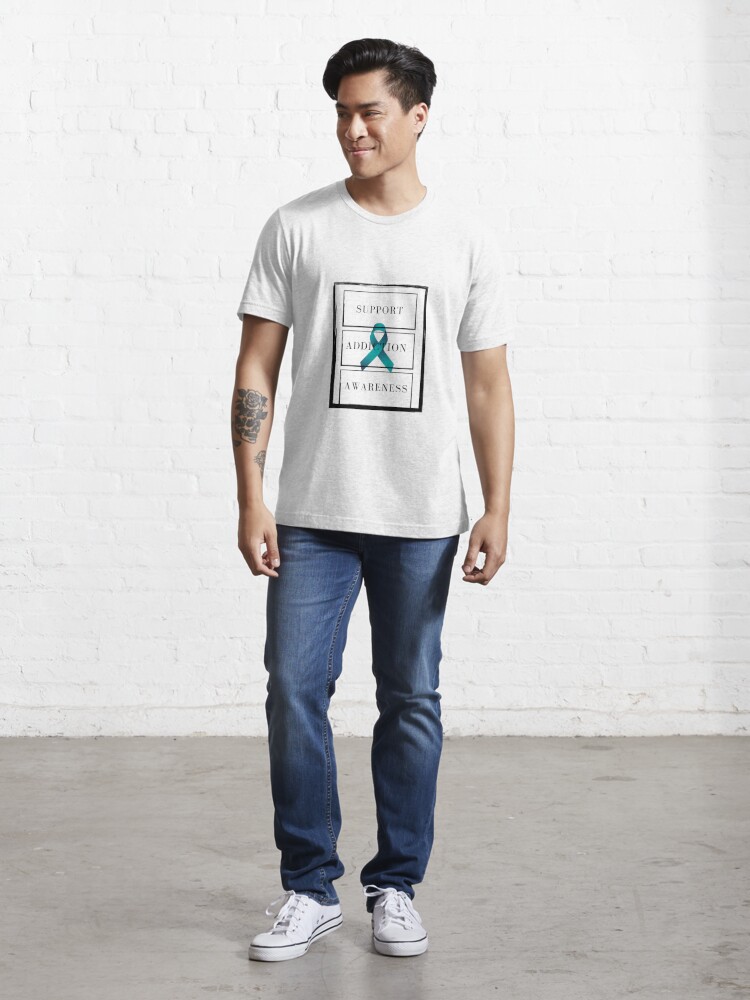This photograph features a man posing confidently in a brightly lit indoor setting with smooth, gray flooring and white painted brick walls. The subject, who has short, poofy black hair brushed back at the top and a clean-shaven angular face, directs his gaze towards his right while displaying a slight smile. He exudes a model-like presence, dressed in a white t-shirt adorned with a prominent green ribbon. Around the ribbon, the shirt bears the text "Support, Addiction, Awareness" encased in a black rectangular outline. The man also wears blue jeans and white Converse shoes, and has a visible tattoo on one of his arms, adding a touch of personal flair to his look.